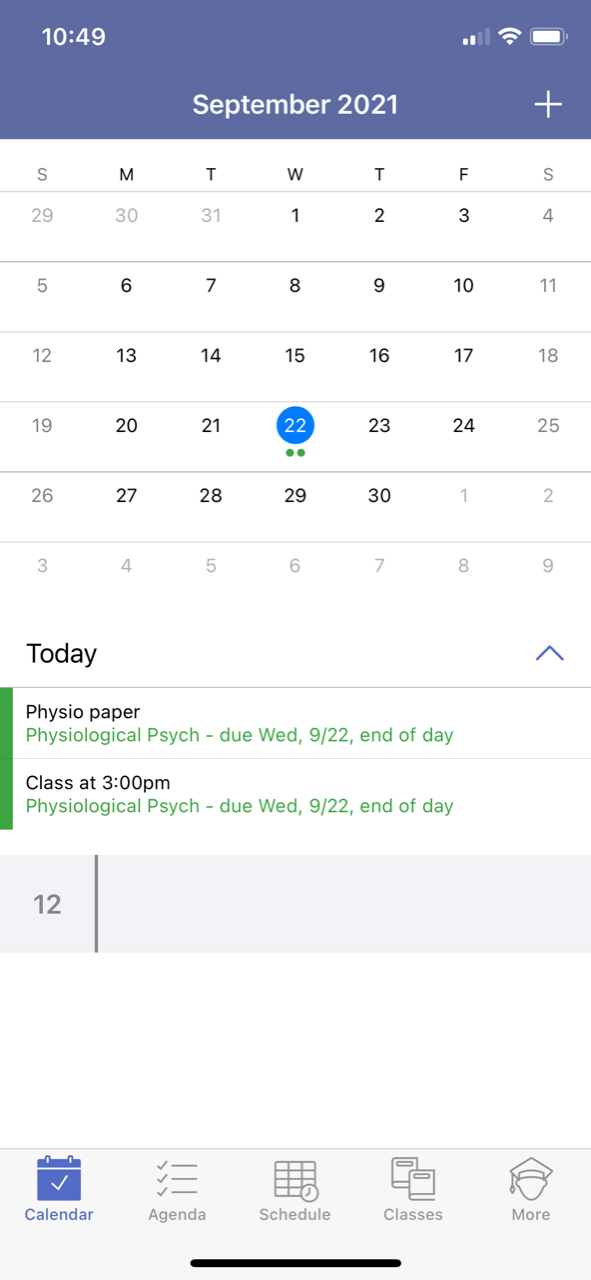This is a screenshot of a calendar app on a phone, specifically displaying September 2021. The header of the calendar is highlighted in purple and prominently features "September 2021" at the top center. In the top left corner, the time reads 10:49, and in the top right corner, there is a battery icon. On the right side, there's a plus sign for adding new events.

The main calendar area has a white background and organizes days from Sunday to Saturday. The month starts on a Wednesday. Notably, September 22 is encircled in blue with two green dots underneath it, indicating events or tasks on that day.

Below the calendar, there's a section titled "Today." This section is divided into two rows. The first row contains "Physiopaper," and directly below it in green text, it says, "Physiological Psych, due Wednesday, 9/22, end of day." The second row lists "Class at 3 p.m.," with the same green text note underneath repeating, "Physiological Psych, due Wednesday, 9/22, end of day."

At the bottom footer of the app, there are five icons representing different functionalities: Calendar, Agenda, Schedule, Classes, and More.